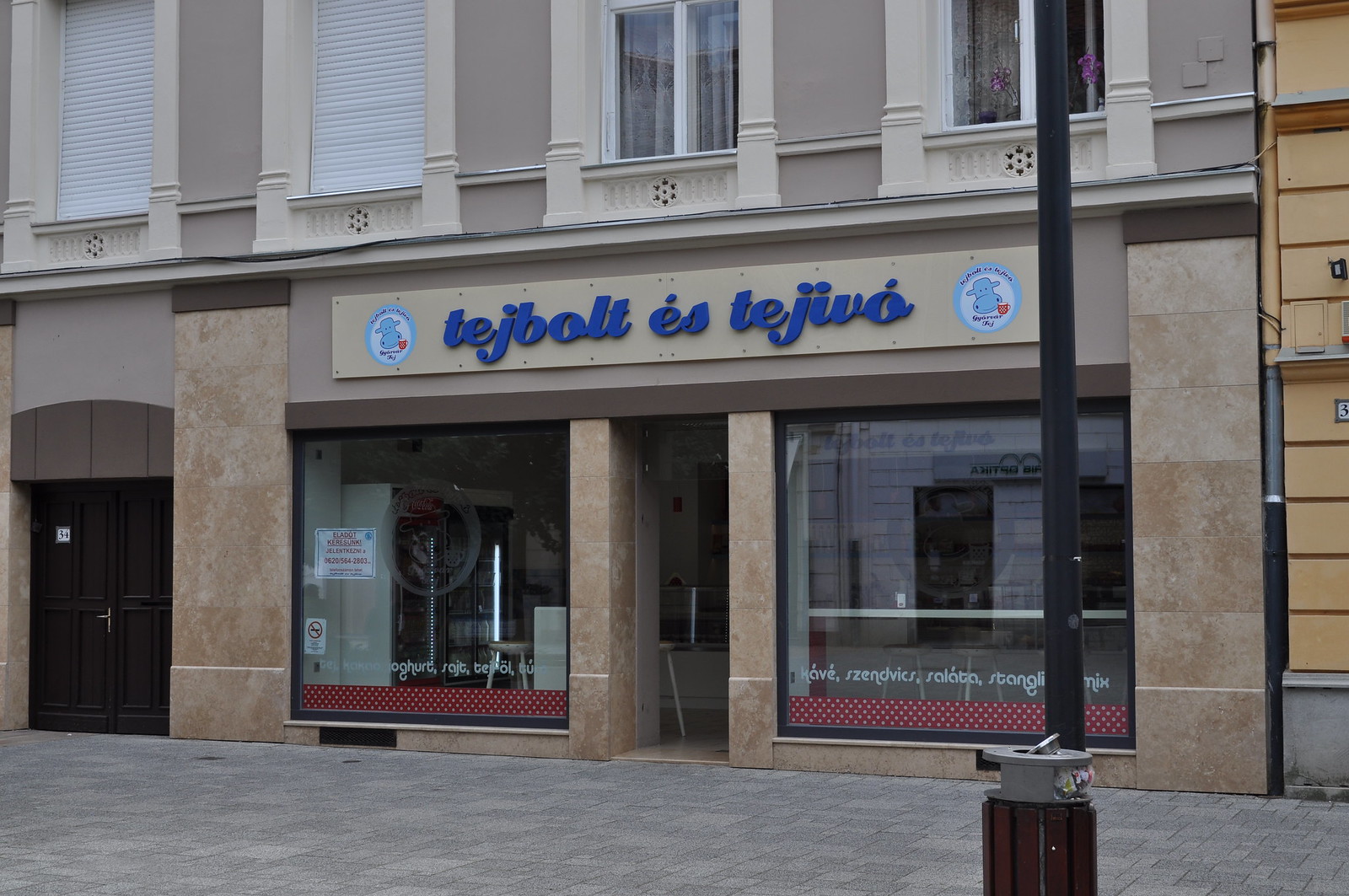The image depicts a quaint storefront situated on a well-maintained cobblestone street in an urban center. Above the storefront, there are apartment windows, some with off-white stone trim and adorned with white blinds or tan curtains, indicating it's part of a multi-story building. The storefront features a prominent blue sign with text that’s not in English, possibly reading "Tejbolte Estegivo," suggesting it might be in Hungarian. Below the sign, there's a whimsical cartoon illustration of a cow and a cup of coffee, hinting that the store might be a café offering items like sandwiches and yogurt. The building facade is a mix of tan stone and features two large windows with red ribbon markings at the bottom and white text on them. Above the entryway and windows, there are two circles with blue and white designs. The entryway itself is flanked by two dark-colored doors to the left. On the bottom right of the frame, there's a silver and black garbage can, and nearby, a street sign and a street lamp mark the urban setting. The photograph appears to be taken from directly across the street in the middle of the day, capturing the bustling yet serene essence of city life.